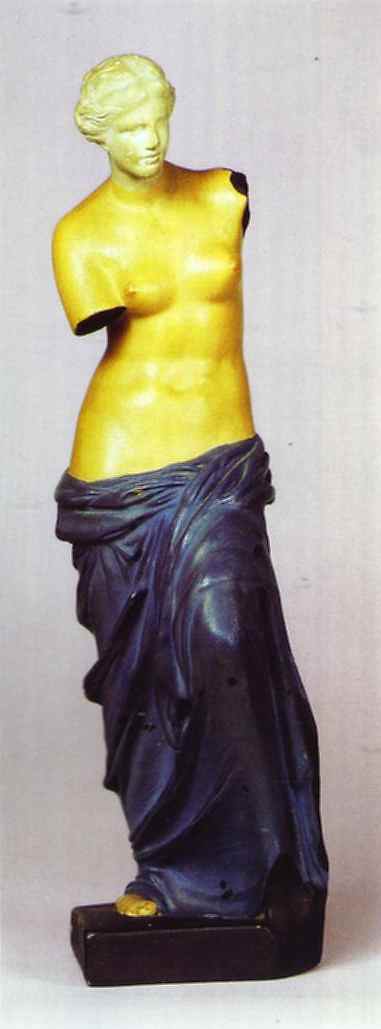The image depicts a marble statue of a woman, approximately two feet tall, against a white wall atop a white surface. The statue features a yellow hue and portrays a female figure with her hair pulled back. Her upper body is unclothed, revealing her torso and breasts, while a dark blue draped garment covers her from below the torso to her feet, with one yellow foot visible poking out from underneath the garment. The statue's right arm is broken off halfway down, and the left arm is missing entirely, severed at the shoulder. The woman stands on a black base.